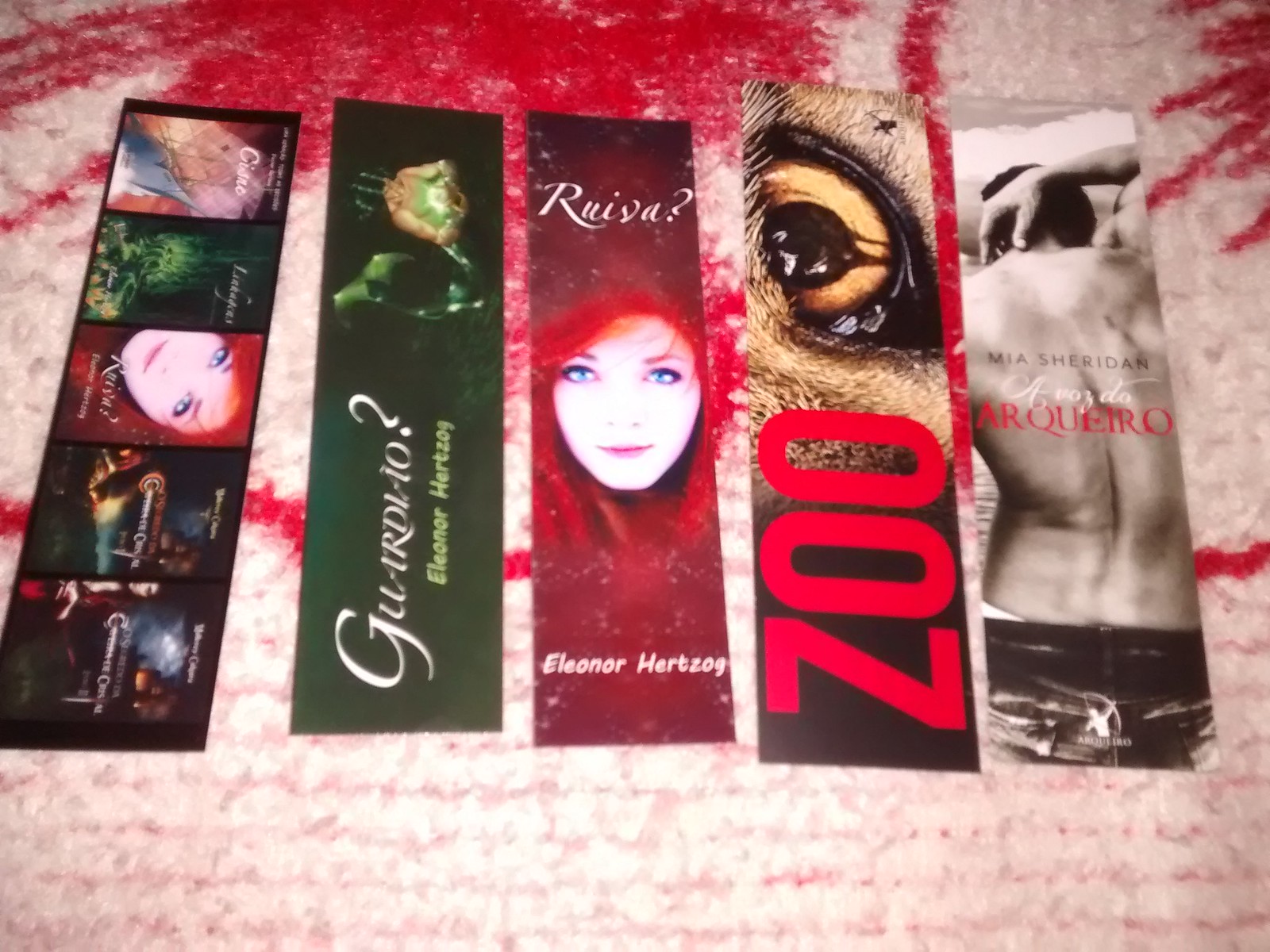This image showcases five rectangular paper bookmarks arranged on a pink and reddish woolen blanket. The bookmark on the far left features five book covers depicted on it. The second bookmark from the left displays the back of a shirtless man scratching his back. In red text, it reads "Mia Sheridar, a voice of an aquarist." The middle bookmark prominently shows the face of a blue-eyed girl with red hair, wearing a red hood, with the text "Riva?" written above. The fourth bookmark to the right depicts a close-up of a golden eye belonging to a wild animal, with the word "Zoo" written in red beside it. The bookmark on the far right reads "Guardiao Eleanor Herzog" in green and white text. All bookmarks are placed neatly on a beige fabric adorned with red designs.